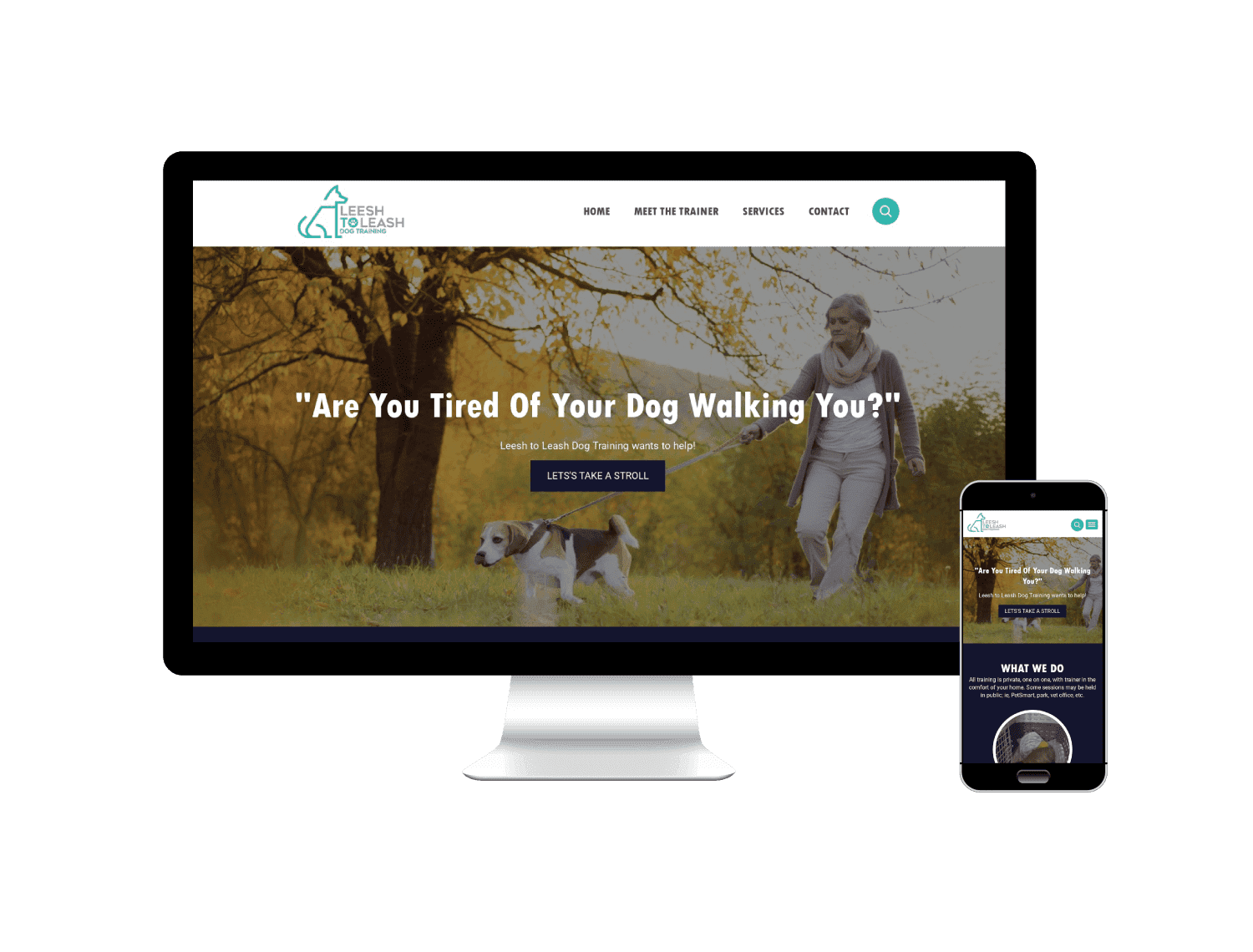A screenshot of a computer display captures the homepage of a dog training service named "Leesh to Leash Dog Training." Prominently displayed at the top is the company name, where "Leesh" is creatively spelled "L-E-E-S-H" and "Leash" is spelled "L-E-A-S-H," accompanied by an illustrated, teal-colored dog. Navigational options, including "Home," "Meet the Trainer," "Services," and "Contact," are set against a white background, along with a teal circle encompassing a white magnifying glass icon.

The main foreground of the image features the bold question, "Are you tired of your dog walking you?" followed by the statement, "Leesh to Leash Dog Training wants to help." A black button at the bottom says, "Let's take a stroll."

In the background, a photograph shows a determined Beagle forcefully pulling on its leash, causing a slight choke. The dog’s tongue is visible, signaling its eagerness. A woman, presumably the dog's owner, attempts to keep up. On the right side of the screen, a mobile phone display shows the same image and includes a section titled "What We Do."